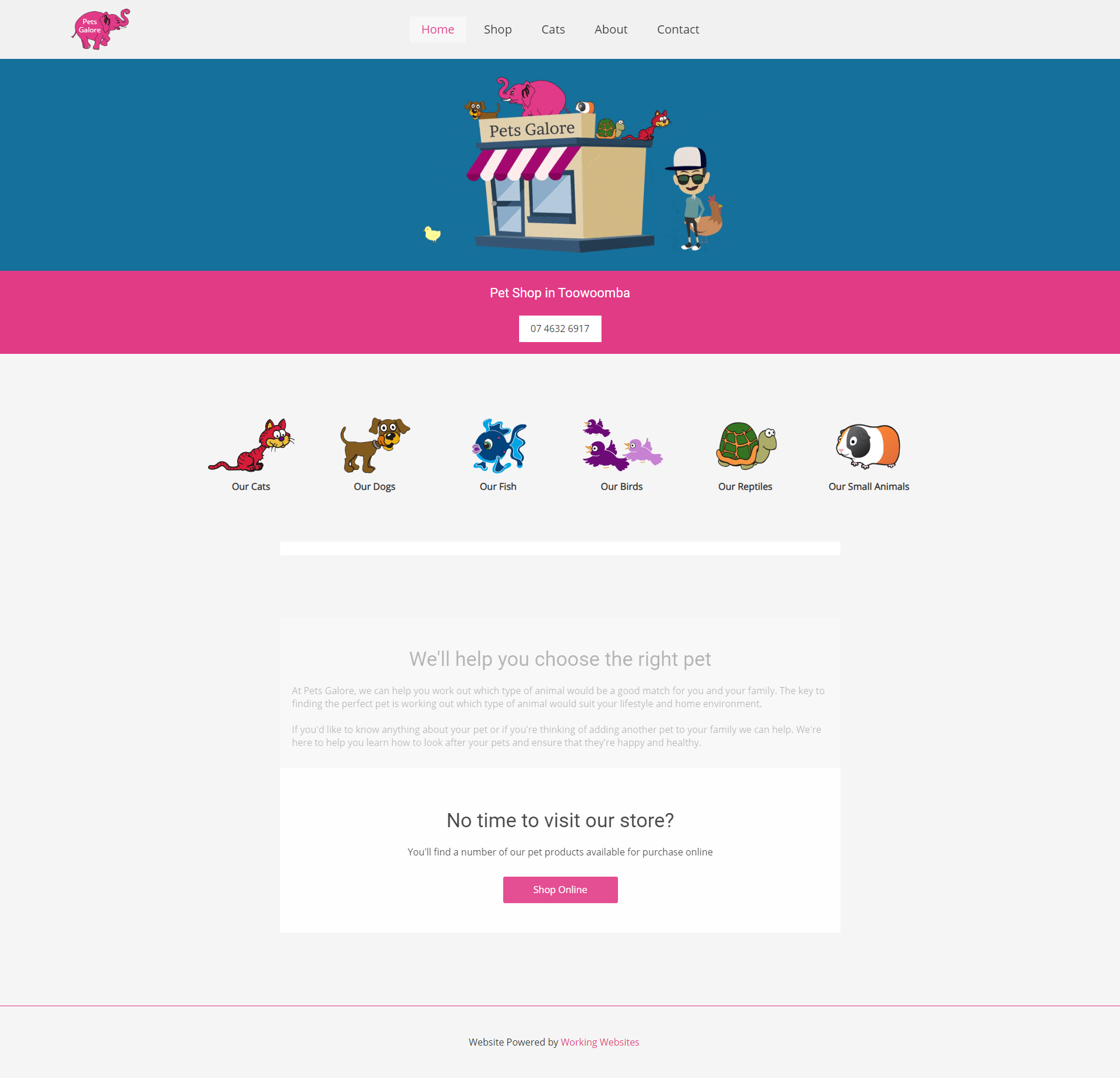**Detailed Caption: Screenshot of Pet Store Landing Page**

The image depicts a detailed screenshot of the landing page for a pet store named "Pets Galore." At the top, there is a navigation bar with a gray background featuring a distinguishable brand icon of a pink elephant with the store's name, "Pets Galore," in white text superimposed on the elephant's body. The elephant's trunk is oriented to the right. 

In the center of the navigation bar, five options are displayed: "Home" (which is currently selected and highlighted in pink text against a nearly white background), "Shop," "Cats," "About," and "Contact" (all shown in gray and unselected). 

Below the navigation bar, a larger blue bar spans the width of the page, showcasing a cartoon illustration of the "Pets Galore" storefront. The store's name is also displayed here, with an elephant on the roof accompanied by other pets including a dog, a turtle, and a cat. The storefront features a fabric awning with purple and white diagonal stripes, one door, and one window. To the right of the store stands a cartoon man wearing a white and black baseball hat and sunglasses, with a chicken behind him. A baby chick is positioned to the left of the store.

Immediately beneath this blue section is a hot pink bar featuring the central text "Pet Shop in Tu Wumba," accompanied by a light gray rectangle displaying the numerals "07 4632 6917."

Further down, the bottom portion of the page presents six cartoon icons representing different types of pets, each with a playful color scheme: 
- Cats (orange)
- Dogs (brown)
- Fish (blue)
- Birds (three birds flying to the left, with the leftmost two in purple and the rightmost in light pink)
- Reptiles (a green turtle with yellow shell accents)
- Small Animals (a gerbil or hamster colored with orange, white, and black)

In the center of this section, a grayed-out text box reads "We'll help you choose your pets," followed by two lines of fine print and then another two lines of fine print.

Below this, a lighter background box states, "No time to visit our store?" This is followed by smaller text that reads, "You'll find a number of our pet products available for purchase online," with a prominent pink action button labeled "Shop Online."

Towards the bottom of the page, there is a thin dividing line in purple or pink, with the very bottom of the page displaying the text "Website powered by" in pink, centered above the phrase "Working Websites."